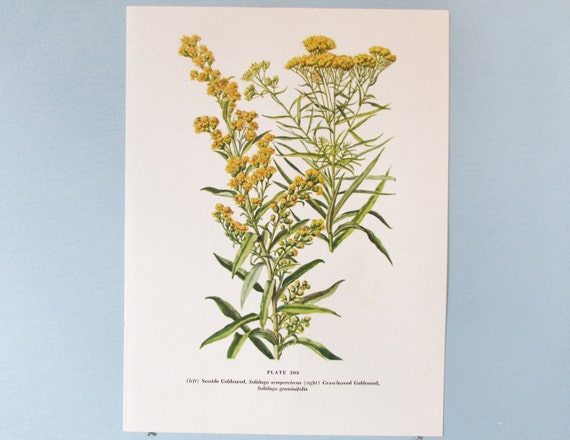This image showcases a detailed botanical artwork mounted on a pastel blue wall. The artwork, drawn on a white piece of paper, features an intricate representation of a plant with a slender green stem, lined with delicate leaves. The focal point of the drawing is the cluster of yellow flowers, some fully bloomed while others are only budding. Additional illustrations offer a more zoomed-out view of the plant, highlighting more of the stem and foliage, with sharp, pointy leaves. Both versions of the plant’s depiction are accompanied by a block of purple text, which is unfortunately too blurry to decipher. The paper is affixed to the wall using two visible fasteners at its bottom corners, giving it a scientific illustration feel reminiscent of images found in old botanical encyclopedias.